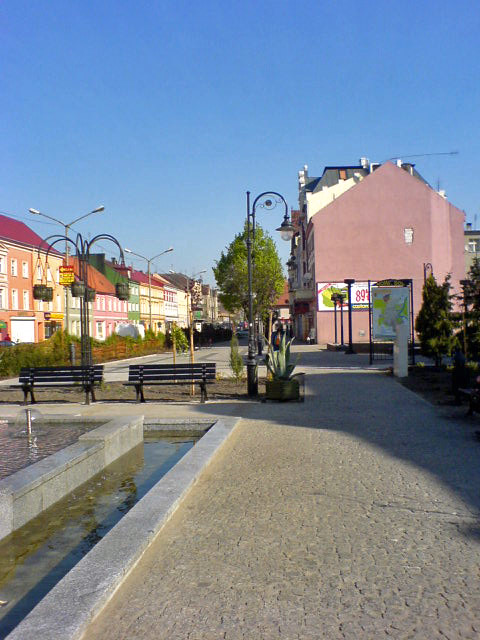The image depicts a lively city square bathed in sunlight under a clear blue sky. In the foreground, a gray stone walking path meanders through the scene, initiating from a fountain in the bottom left corner. The fountain, made of blue and gray hues, features water elegantly streaming out in an umbrella fashion from a concrete basin. Flanking the fountain are two green benches, oriented to face the flowing water, accompanied by a few black street lamps above them.

The stone pathway divides the image, with the right side leading to a salmon-colored building. Adjacent to it on the left stands a verdant tree, creating a natural balance against the urban backdrop. As the path extends towards the center, it introduces a lineup of vibrant, closely-knit buildings of various colors—orange, yellow, green, red, and kelly-green—each adding a splash of life to the scene.

Above these residences, a poster on a building, faintly displaying the number '89,' indicates a market-like atmosphere, perhaps hinting at local produce. In contrast to the bustling lower half, the top half of the image opens up to a serene and expansive light blue sky, framing the picturesque downtown area that exudes a blend of residential charm and tourist appeal.